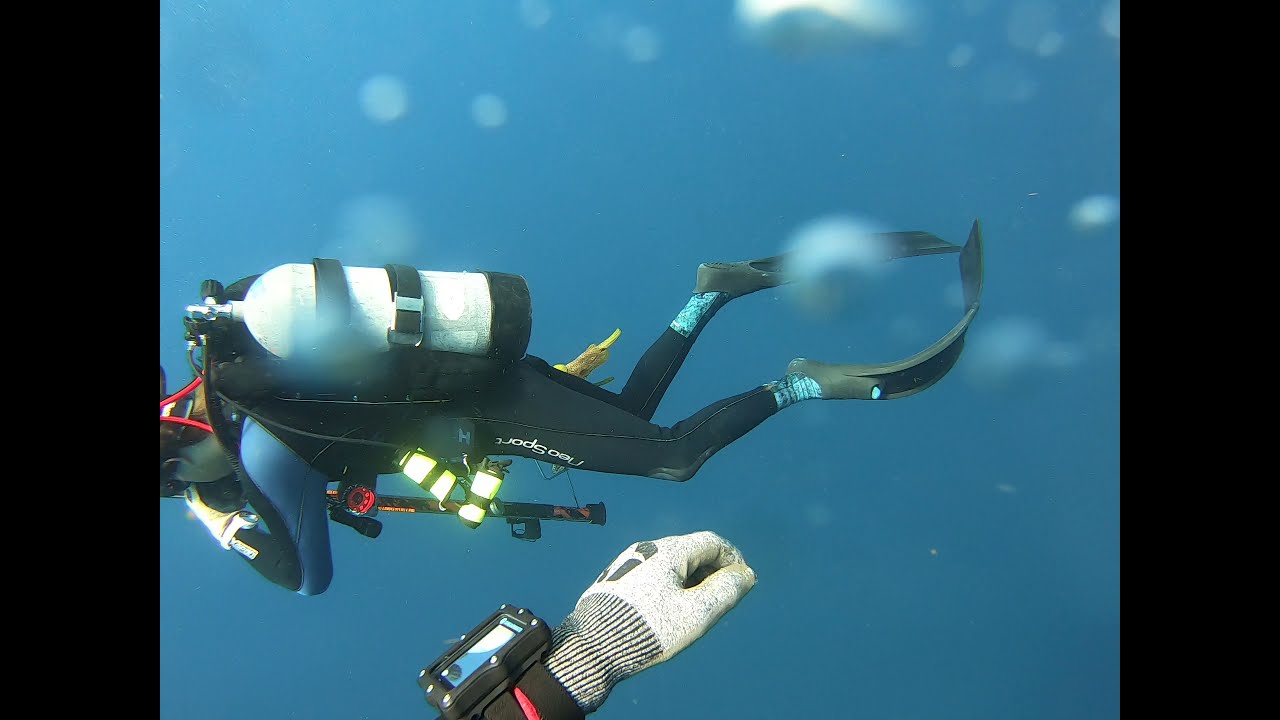In this underwater photograph taken in the ocean, the vibrant blue water creates a calming backdrop, speckled with bubbles that gently blur parts of the image. At the bottom, a hand wearing a beige glove and equipped with what appears to be a dive meter or GPS is visible, likely belonging to the photographer. This hand, around which red cords can be seen, suggests the person might be wearing a red wetsuit. Centered in the image is another scuba diver swimming horizontally. This diver is clad in a black wetsuit with blue accents, wearing gray flippers and managing breathing equipment, possibly an oxygen tank and additional canisters attached to the waist. The scene feels dynamic and immersive, capturing the essence of an underwater adventure.